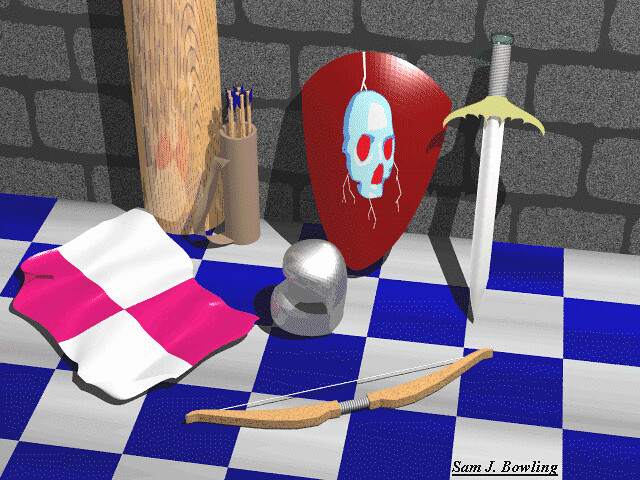The image is a pixel art drawing showcasing an array of medieval-style equipment against a backdrop of a gray brick wall and a blue-and-white checkerboard floor. Dominating the scene, slightly left of center, is a damaged, rectangle-shaped shield adorned with large red and purple checkerboards on each diagonal side, appearing creased and bent. To its right lies a simple silver knight's helmet with its opening pointed left, and next to it, a quiver of arrows with blue fletchings. Central to the image, a striking red shield featuring a white skull with red eyes and a nose opening stands against the wall, slightly covering a thick natural wooden post. Further right, a silver sword with a yellow, wide flanged handguard and a green handle rests against the wall, its tip touching the floor. Below these is a simple wooden bow, with its string oriented towards the background. In the far left corner on the floor is a pink and white checked flag, positioned diagonally. Additionally, faintly visible on the wall is a delicate painting of a woman in a dress with a sweater beside a brown lever and a cylinder holding extra-long wooden matches. The text “Sam J. Bowling” is underlined and displayed in black at the bottom right of the image.